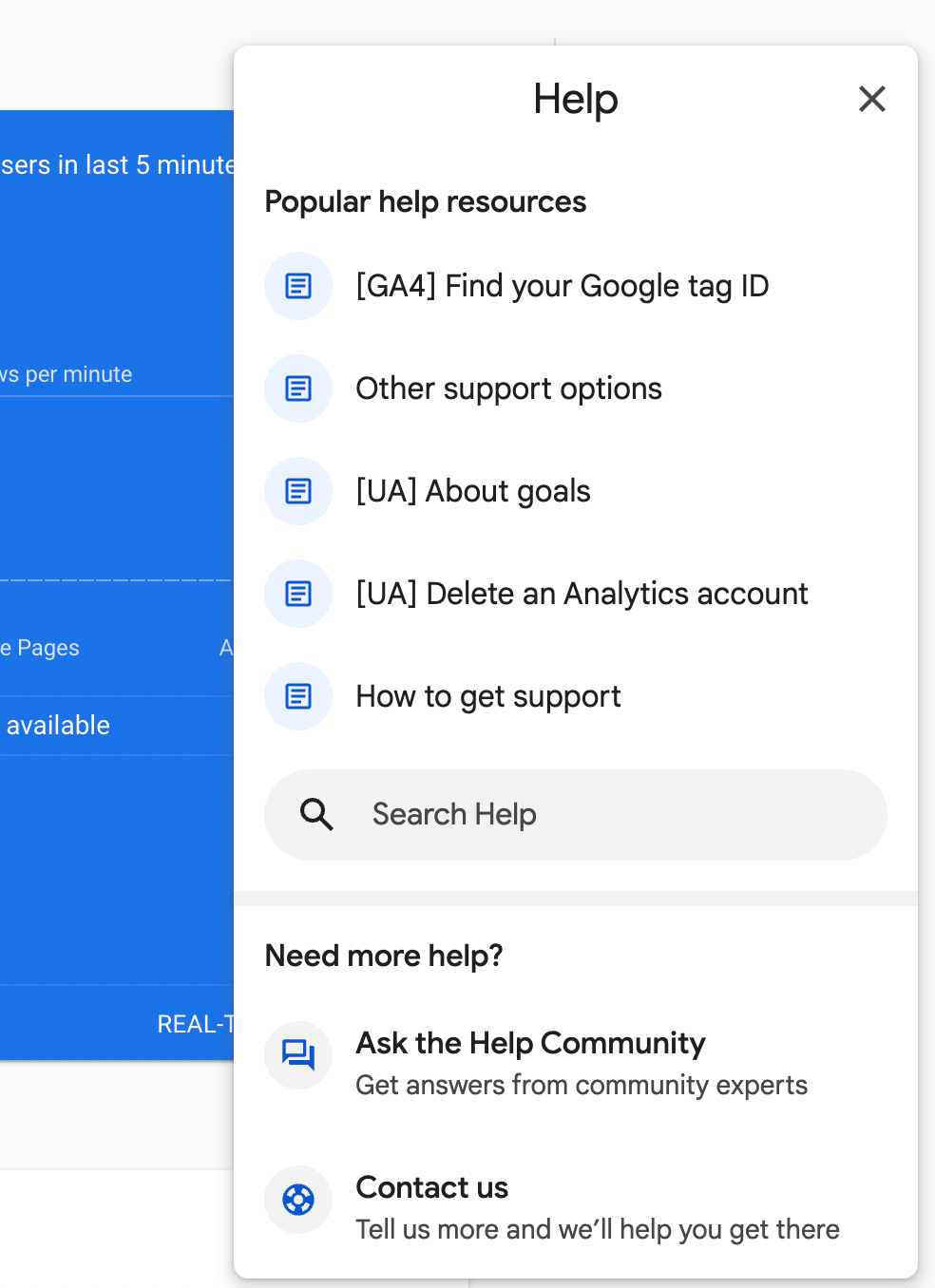This detailed screenshot captures a tooltip menu designed to provide help resources. The tooltip is characterized by a sleek, white, rounded-rectangle shape, oriented vertically. At the top of the menu, the heading "Help" stands out prominently, with a close button (an 'X' icon) situated in the top-right corner for easy dismissal.

Below the heading, the menu features the subheading "Popular Help Resources," under which five help topics are listed. Each item in the list is accompanied by a blue circular note icon, enhancing visual identification. The topics are:

1. GA4: Find Your Google Tag ID
2. Other Support Options (UA)
3. About Goals (UA)
4. Delete and Analyze Account
5. How to Get Supported

At the bottom of the tooltip, there is a functional search bar labeled "Search help," complete with a magnifying glass icon on its left side, allowing users to search for additional help topics.

Overall, the easily navigable layout and clear headings ensure that users can quickly find and access the support information they need.